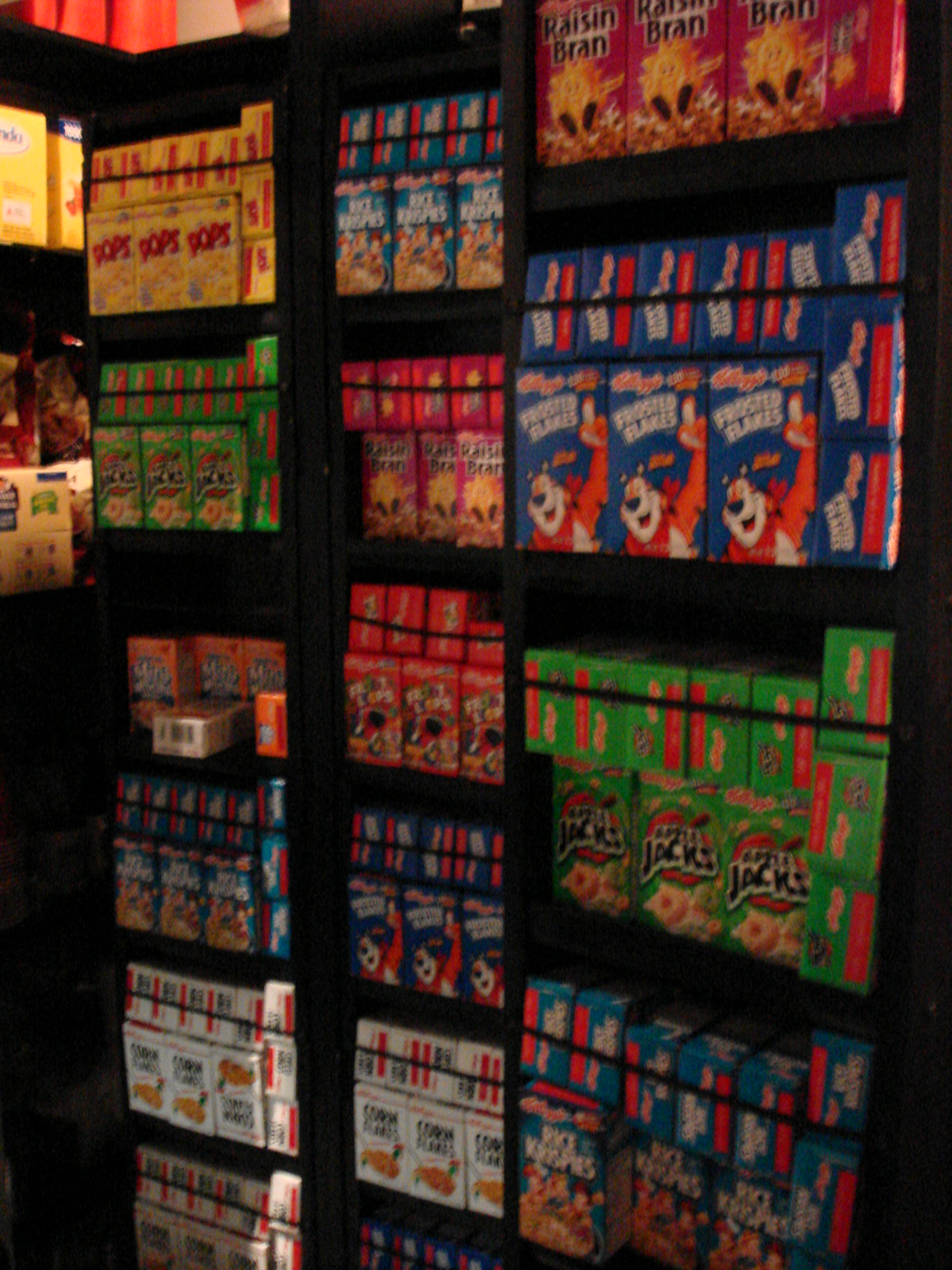This photograph captures a detailed view of a cereal display inside a small store, possibly a bodega or convenience store. Dominating the center are three tall, open-faced shelving units, each reaching about six feet high and divided into six shelves. The display units are black, possibly made of dark wood or plastic. The middle and right shelving units appear slightly larger than the one on the left. The shelves teem with an array of brightly colored cereal boxes, neatly stacked and grouped by type. Featured cereals include Corn Pops, Apple Jacks, Rice Krispies, Corn Flakes, Frosted Flakes, and Raisin Bran, with some shelves showcasing smaller, likely single-serving boxes, especially on the left unit. The rightmost shelf stands out with its broader sections, holding larger cereal boxes. In the background, partially obscured, is another black shelving unit displaying items that look like oatmeal and grits. The scene suggests a well-organized, inviting setup meant to catch the eye of shoppers, emphasizing the variety and abundance of breakfast options available.